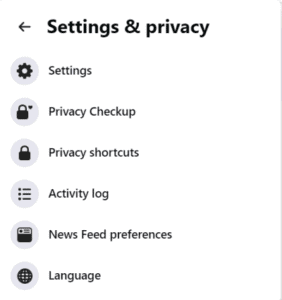This is a detailed description of a screenshot depicting a settings and privacy menu from an unspecified application. At the very top of the menu, the title "Settings and Privacy" is displayed, accompanied by a left-facing arrow on the far-left side of the screen, indicating a navigation option to return to the previous screen. Below the title, the menu options are vertically arranged, each icon enclosed in a gray circle and the icons themselves rendered in black against a white background. 

The first option is represented by a gear icon labeled "Settings." Following this is a lock icon labeled "Privacy Checkup," another lock icon for "Privacy Shortcuts," three vertical dots with lines next to them labeled "Activity Log," an icon resembling a newspaper labeled "News Feed Preferences," and lastly, a grid-like world icon labeled "Language."

On the right side of the screen, a vertical gray line runs the length of the menu. The black text on a white background enhances readability while the narrow, vertical orientation of the screenshot suggests it is likely captured on a mobile device. However, there is no additional context provided to ascertain the specific application or platform from which this menu originates.